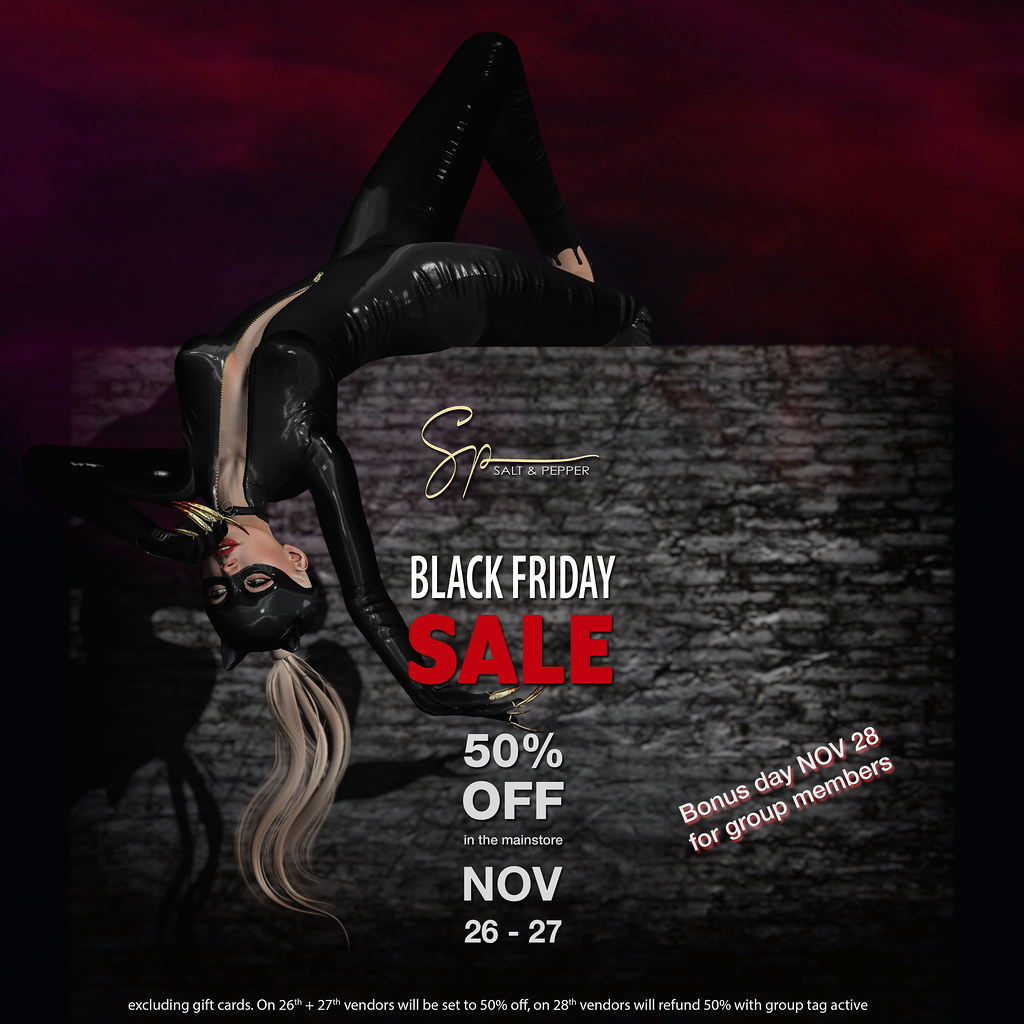This striking advertisement for Salt & Pepper’s Black Friday sale features bold text at its center, with "Black Friday" scripted in white and "SALE" in a prominent red font. Below this, “50% off” is displayed in white, with the sale dates, November 26-27, clearly indicated. An additional note in a slanted upward print reveals a bonus day on November 28 for group members. The image backdrop is composed of a gray, old-style brick wall, likely a facade, which contrasts sharply with the rest of the dark-toned image. Dominating the left side of the visual, a woman dressed in a shiny, black polyurethane catsuit reminiscent of Catwoman is dramatically posed. Her bodice, unzipped to her navel, suggests a provocative allure. She reclines backward over the wall, her upper body hanging upside down with her face masked and only her eyes visible, framed by striking, very red lipstick. Her long, blonde ponytail cascades down, while her one leg is bent at the knee, exposing the full length of the catsuit which extends to her ankle. The background features subtle shades of blue, red, and purple, adding depth to the dramatic scene. At the bottom of the advertisement, a small note informs customers of a special condition: excluding gift cards and a refund of 50% on November 28 with an active group tag. The entire visual is designed to captivate and draw attention to the 50% off sale, urging viewers to join in on the lucrative Black Friday deals.